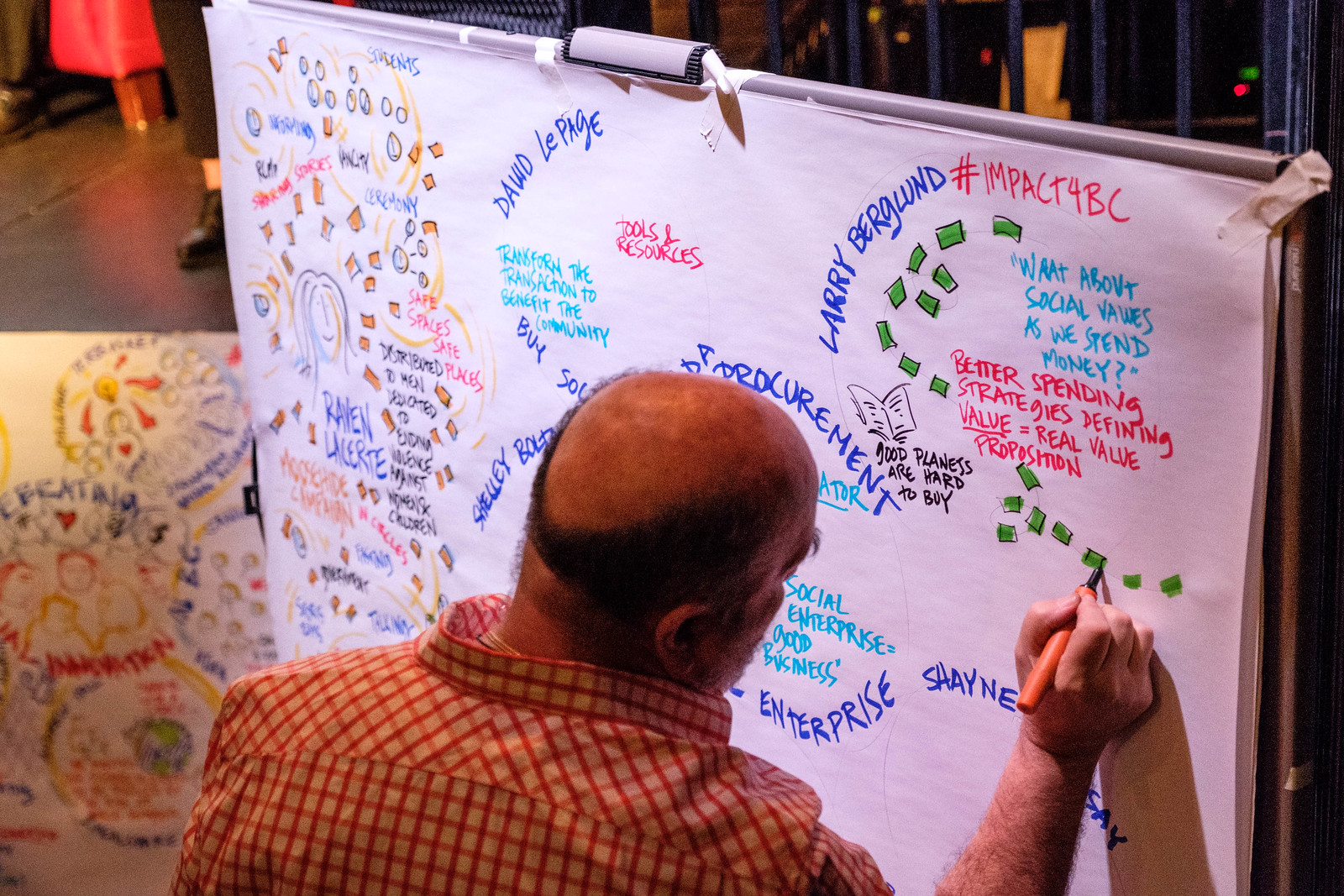The image depicts the back of a bald man who is actively engaged in a drawing session at an easel holding a large pad of paper. He is wearing a collared, red-and-white checkered shirt and using a thin-tipped marker, specifically a green sharpie, to add to the detailed and colorful artwork on the page. The scene appears to be set in an indoor workshop or brainstorming session. The pad is covered with neatly written text and various artistic illustrations, including names like David LaPage, Skelly, and Shane, along with terms such as "procurement," "enterprise," and "better spending strategies." There are also depictions of small dollar bills and phrases like "tools and resources" and "transform the transaction to benefit the community." Words like "defining value equals real value" and "good plans are hard to buy" are prominently featured. In the background, part of a wooden floor is visible along with someone’s legs and feet, as well as some additional papers and a gate. The photo is taken from an elevated angle, providing a comprehensive view of the man's activities and the setting.